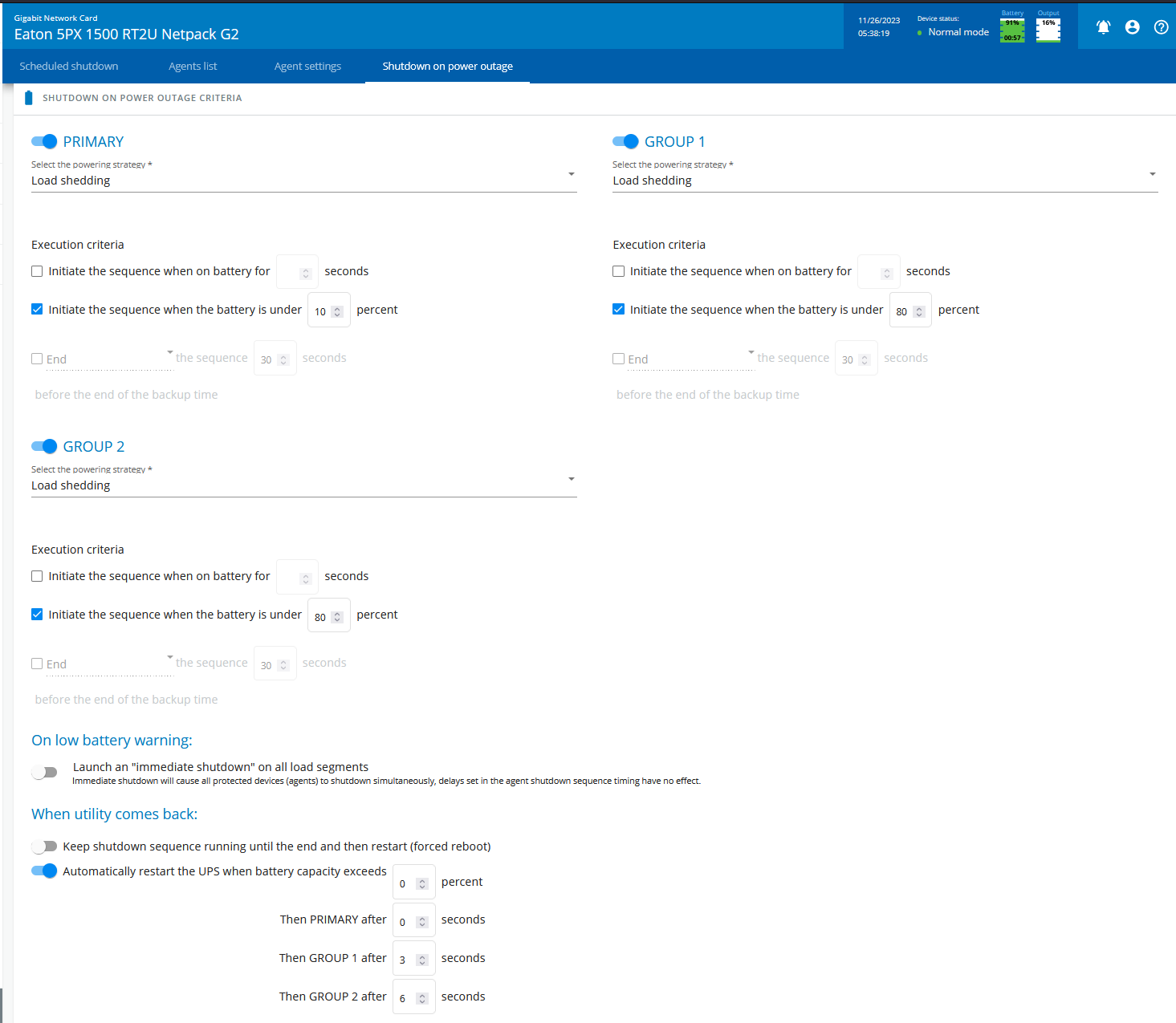The image is a detailed screenshot of a computer interface, likely from a management console for an Eaton UPS system. The interface contains extensive information, primarily focused on the UPS's status and configuration settings. Key details include:

At the top of the screenshot, on a lighter blue banner, the text "Gigabit Network Card Eaton 5PX1500RTT2U NetPack G2" is displayed. To the right, the current date and time "11-26-23 at 5:38:19" is visible, along with the device status showing "Normal Mode." The battery is indicated to be at 91%. Below this, the values "00.57" and "Output is 16%" are recorded. The battery icon shows a nearly full green bar with a small white sliver at the top, while the output icon shows a predominantly white bar with a small green sliver at the bottom.

On the right-hand side, there are several icons for notifications, user account, and help (question mark in a circle). The main navigation options across the interface read "Scheduled Brick Shutdown," "Agents List," "Agent Settings," and "Shutdown on Power Outage." The last option is highlighted in white and underlined, indicating it is the current active section.

The "Shutdown on Power Outage" section features a white background with the header "Shutdown on Power Outage Criteria." The "Primary" toggle, indicated in blue to the left, is switched on. The execution criteria listed include:
1. "Initiate the sequence when on battery for [ ] seconds," with an unchecked white square.
2. "Initiate the sequence when the battery is under 10%," which is checked in blue.

The "Group 2" section similarly features a blue toggle, which is on. Options included are "Select the powering strategy" with a drop-down box currently set to "Load Shedding." Execution criteria again have:
1. "Initiate the sequence when on battery for [ ] seconds," which is not checked.
2. "Initiate the sequence when the battery is under 80%," which is checked in blue.

Further details include: 
- "On low battery warning," launch an "Immediate Shutdown" on all load segments, which is not enabled (gray toggle).
- "When utility comes back, keep shutdown sequence running until the end, and then restart (forced reboot)," also disabled (gray toggle).
- "Automatically restart the UPS when battery capacity exceeds [0]%" is enabled with an associated primary action after zero seconds. Group one is set to restart after three seconds, and group two after six seconds.

The upper right corner shows "Group 1," with similar settings and toggles as described, including "Select the powering strategy" (Load Shedding) and execution criteria (like initiating the sequence when on battery for a specified time or battery level below 80%).

Overall, the captured image provides comprehensive data and controls for configuring and monitoring an Eaton UPS system, presented in a technical, user-interactive format commonly used by IT or facilities management professionals.